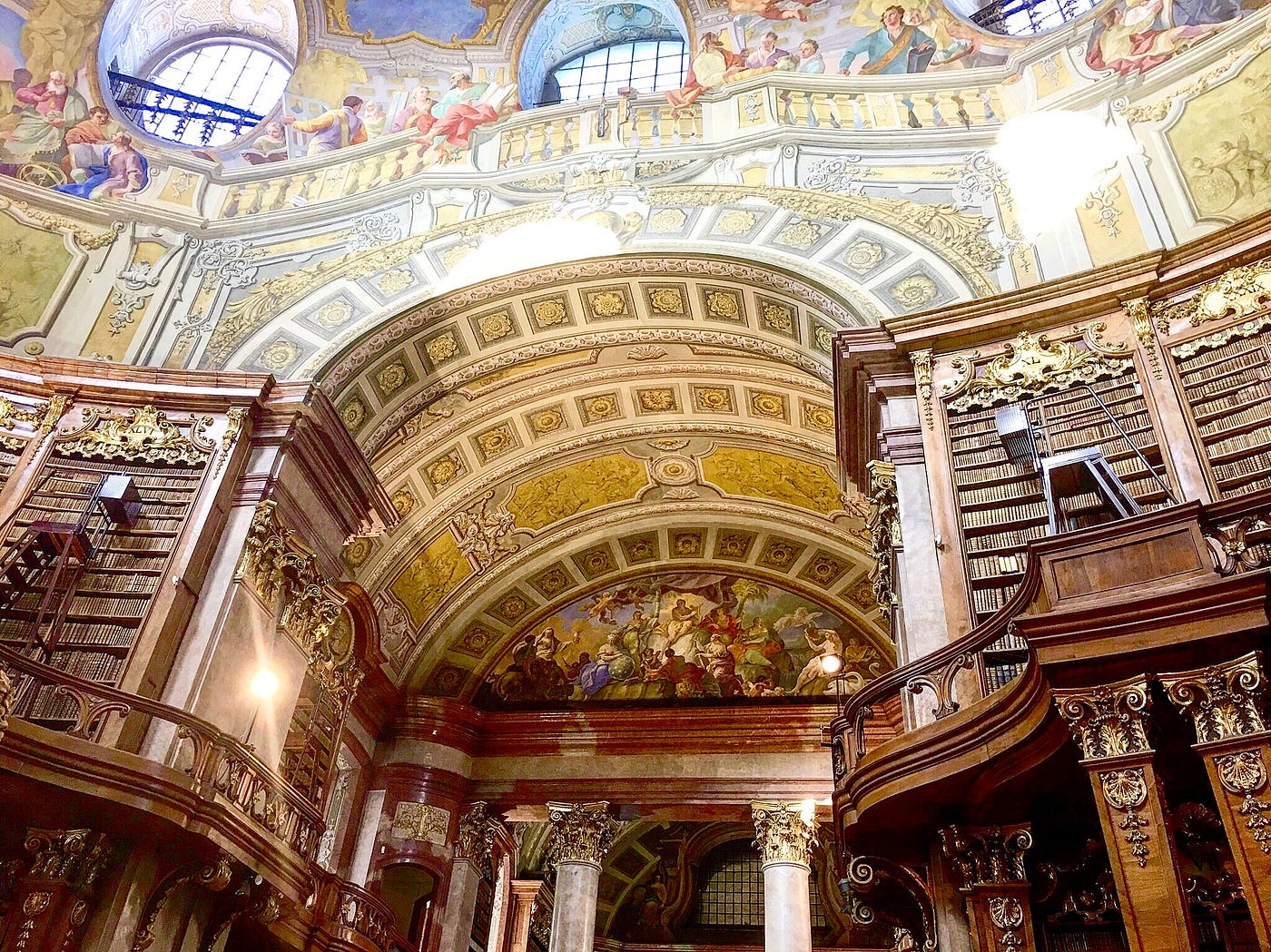The image depicts an opulent interior scene that blends characteristics of a European cathedral and a luxurious library, reminiscent of Renaissance architecture. The focal point is an intricately painted ceiling similar to the Sistine Chapel, featuring vivid artwork of figures dressed in classical attire, likely representing philosophers like Aristotle and Socrates. These paintings seamlessly incorporate three large windows at the top of the scene, filling the space with natural light.

Dominating the scene is a grand archway, richly detailed and painted to emulate marble, with a mix of yellow and brown tones that complement the surrounding wooden bookcases. These bookcases, adorned with intricately carved woodwork and accessible by ladders, line both sides of the image, heightening the sense of grandeur. The wood’s warm hues harmonize with the painted ceiling and the ornate decor.

Below the archway lies a passageway adorned with further paintings and supported by solid white marble columns, showcasing an elaborate mix of materials. Despite the richness of the visible elements – from the opulently painted arch to the ornate woodwork and marble columns – the scene extends into a more mysterious tunnel, hinting at further splendor beyond the immediate view. The overall ambiance is one of artistic excess and historical gravitas, combining the reverence of a cathedral with the intellectual allure of a classical library.